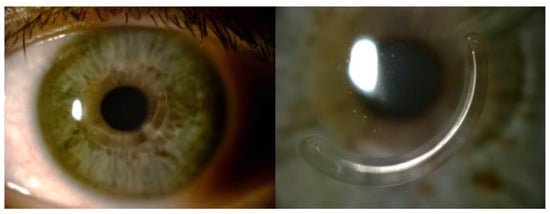The image presents two color photographs of a single human eye in extreme close-up, displayed side-by-side in a landscape orientation. The left photograph showcases a detailed view of the eye, capturing it from the top row of eyelashes down to just above the bottom lashes. The eye features a rich greenish-brown iris surrounded by visible veins within the white sclera. Tiny red spots are noticeable in the corner of the eye, and the pupil is centered and of average size. The background to the right of this eye fades into darkness. In contrast, the right photograph offers an even more magnified view of the same eye, seemingly taken through a special lens treatment, creating a cloudy effect. This second image reveals a dilated pupil and highlights a large white blotch in the left center of the eye, with an arc-like reflective band beneath it suggestive of an implant or medical incision. The surrounding colors transition from whitish gray in the lower zones to darker green in the upper right, contributing to its surreal, almost abstract appearance. Together, these images appear to represent a before-and-after comparison, embodying photographic realism with a representational approach.